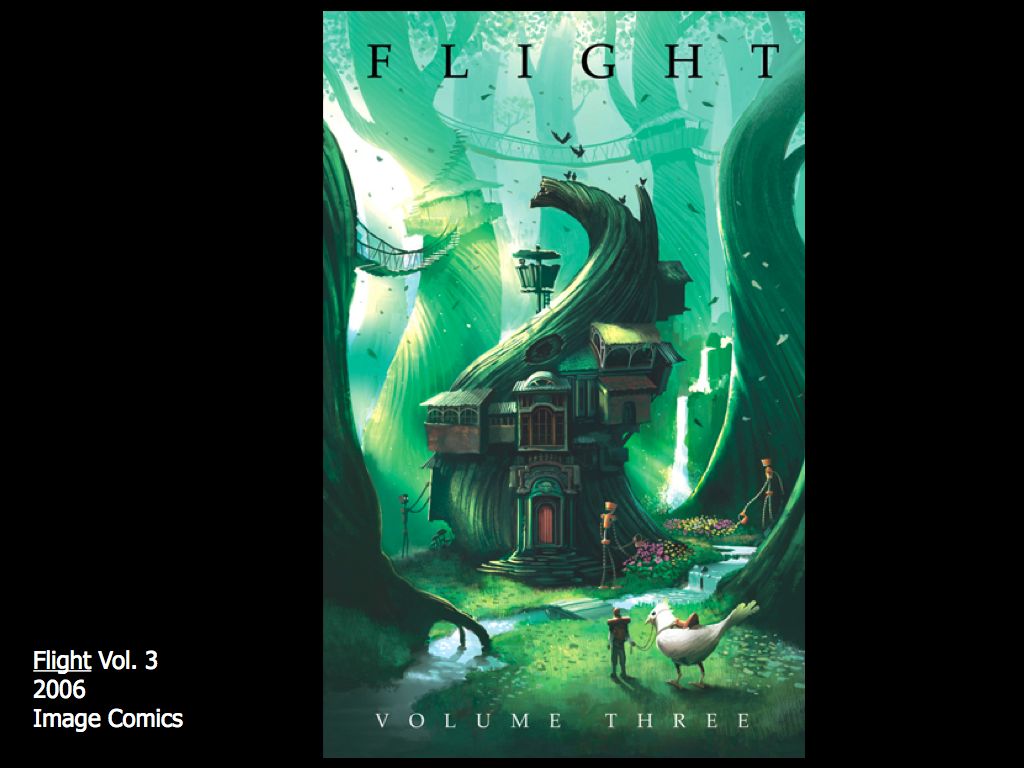The image depicts the cover of a comic book titled "Flight," with the title rendered in a serif, dark font at the top. The issue, identified as "Volume 3," is published by Image Comics in 2006, as indicated in white text at the bottom and side of the cover. The cover is set against a dark background that extends to at least twice the width of the cover, creating ample negative space around the main artwork.

The captivating artwork showcases a fantastical scene at its center. A man leads a large white bird of similar size, guiding it with reins attached to a saddle on the bird’s back. They are headed towards a unique house embedded in a tree. This tree twists upwards into a spiral and features various windows and a door situated higher up its trunk. Surrounding the central tree-house are several other tree-based dwellings linked by walkways and possibly rope bridges.

In the foreground, the detailed illustration includes small robot-like figures tending to the flora around the base of the houses, watering flowers and maintaining the whimsical environment. Additionally, there's a picturesque stream originating from a small waterfall in the background, flowing around the central tree-house with a quaint bridge crossing over it, further enhancing the enchanted forest village setting.